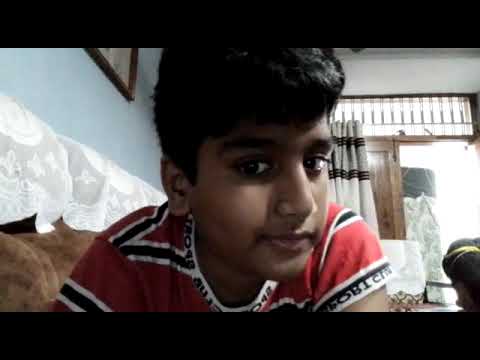In this image, a young boy with thick, dark hair and chubby cheeks is the central focus. He is wearing a red and black short-sleeve shirt with a white outline under the black stripes. Positioned towards the camera, he exhibits a slight rightward turn, offering a semi-half profile view of his face. He is seated on a couch, partially visible in the bottom left of the image, adorned with a doily-like cover. The background reveals a living room setting with a blue wall. There is a framed piece of artwork hanging behind him, and off to the right, a doorway emits a bright light that heightens the overall luminescence. A cream curtain with pin striping is pulled back next to the doorway, through which the light appears to flood in. The position and features suggest a candid, selfie-like photograph intended for social media. The image's color palette includes brown, yellow, white, red, black, and tan.